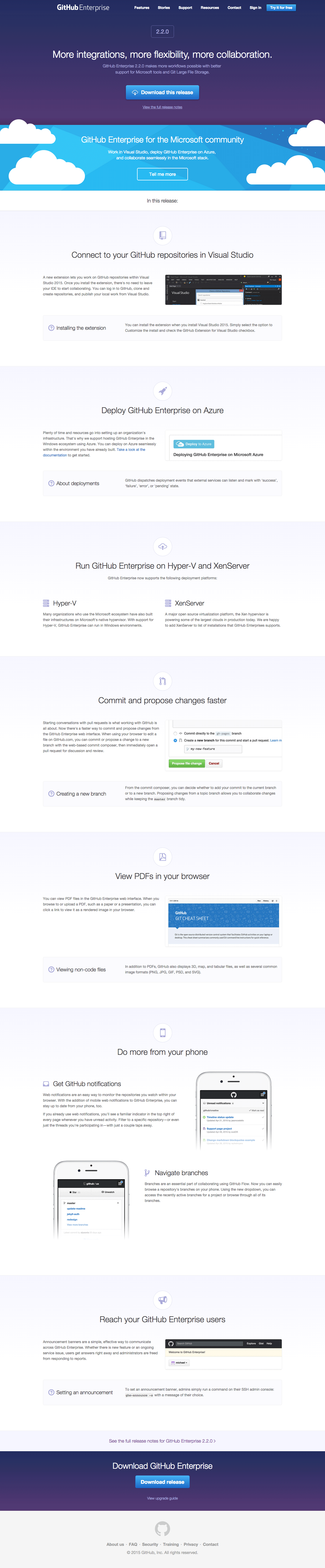Screenshot of a comprehensive website layout captured in a single image. The top section features a navigation menu with a purple background, adorned with white text and a prominent blue button. Below this, a sky-themed section shines with a blue background and white clouds, also containing various white text elements. Following that, the layout transitions into a white-background area segmented into multiple sections. These sections predominantly feature black text, organized into a two-column format. One notable section includes a thin black image positioned on the right side. Another distinct section, entirely composed of text, continues the two-column layout. This repetitive structure creates a consistent and organized presentation throughout the website.